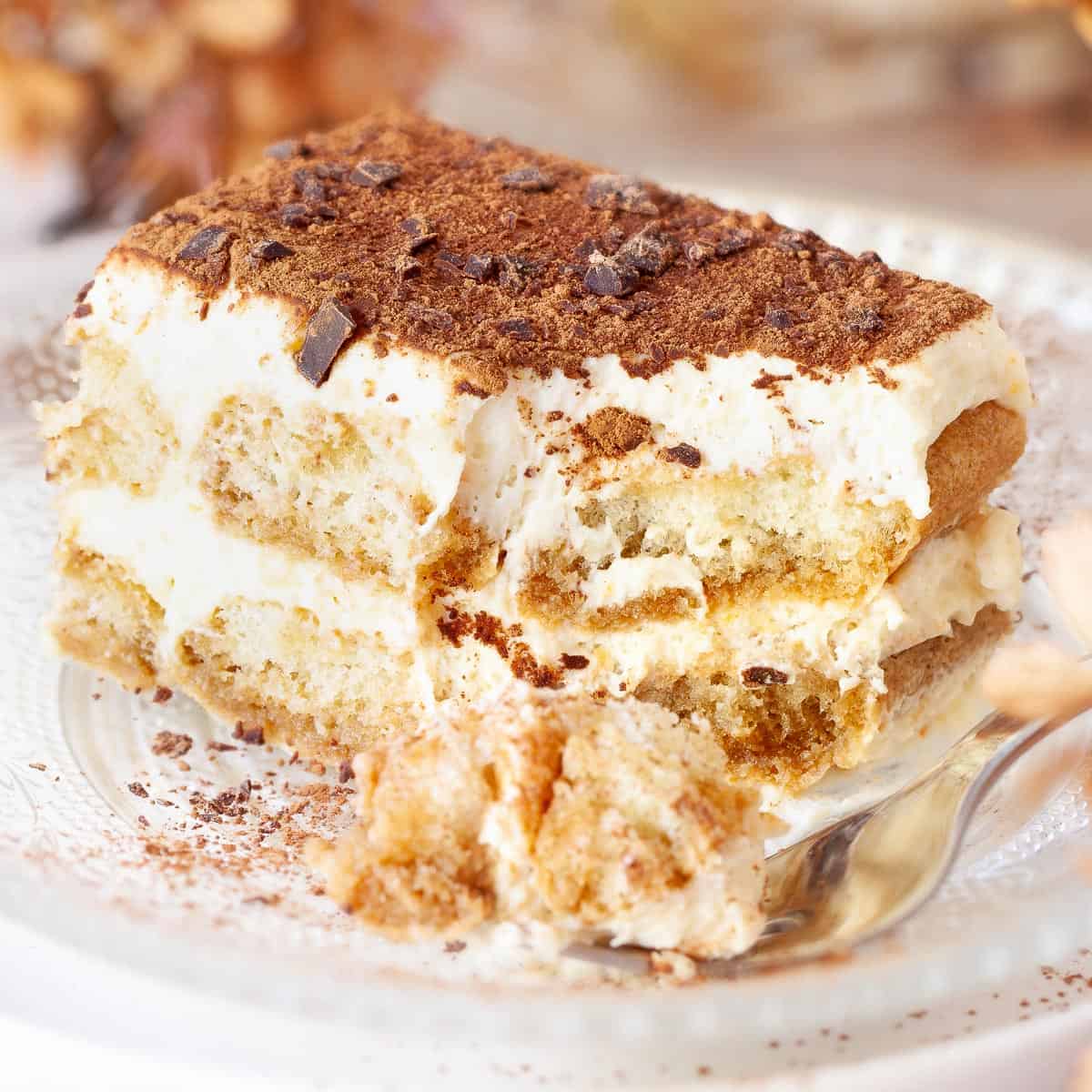An up-close, tantalizing shot captures a plated dessert, possibly taken in a restaurant setting and likely by a food enthusiast. The main focus of the image is a sumptuous piece of cake, appearing to be tiramisu. The dessert is elegantly situated on a white, intricately-indented plate, placed near the front of the frame. A metal fork extends from the right side of the image, showing evidence of a few delicious bites taken. The cake itself is layered meticulously: starting with a sponge cake base, followed by fluffy cream layers, and topped with a rich, chocolate crumble that looks both delicate and flaky. The backdrop is softly blurred, providing a hint of an indoor eating area adorned with warm brown tones and possibly a gray cabinet. The overall scene exudes an inviting ambiance, highlighting the artisanal quality of the cake with its well-defined layers and textures. The dessert's garnishes of chocolate crumbles and perhaps a touch of cinnamon add an extra layer of visual and gastronomic appeal.